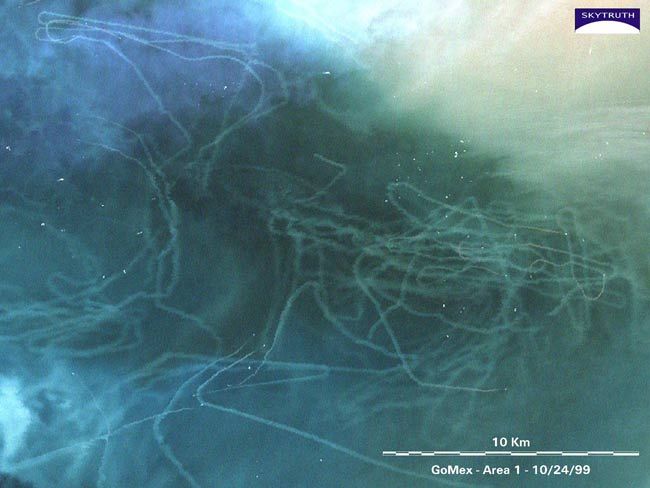A horizontal rectangular image predominantly features a blend of bluish, greenish, and teal hues that merge together, resulting in a hazy, almost abstract appearance. White, wavy squiggles traverse the image, reminiscent of contrails in the sky or strokes in an abstract painting. The upper right-hand corner of the image is slightly brighter, showcasing a small rectangle with a purple background. In white, capital letters, it reads "Sky Truth," accompanied by a white dome shape beneath it. Additional text in the bottom right-hand corner displays "10 kilometers" above a scale line and "Go Max Area 1, 10/24/99," all set in a sans-serif font. The mesh of colors and intricate details give the image an underwater or otherworldly quality, blending art and possibly scientific representation.